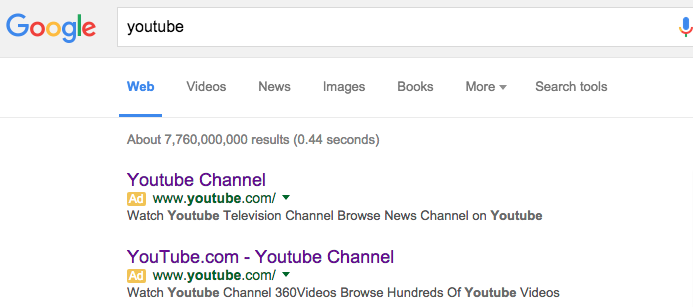The image showcases the results page of a Google search. At the top left corner of the page, there is the iconic Google logo: a capital 'G' in blue, a lowercase 'o' in red, another lowercase 'o' in yellow, followed by a lowercase 'g' in blue, 'l' in green, and 'e' in red. Right next to the logo is the search bar, inside which the term "YouTube" is typed. On the far right inside the search bar is a microphone icon.

Directly below the search bar is a row of tabs. The first tab, highlighted in blue, indicates "Web". The remaining tabs are in a light grayish black color and labeled as "Videos," "News," "Images," "Books," "More," and "Search tools." 

Beneath the tabs, in small gray letters, it reads "About 7,760,000,000 results (0.44 seconds)." Following this, the first search result appears. The main link is in purple and says "YouTube channel." Below this, there's a yellow box with white letters that spell "Ad," and next to it, in green letters, it says "www.youtube.com." Further down in black text, it reads "Watch YouTube television channel, browse news channel on YouTube."

The next entry is similar. The headline is in purple and says "youtube.com - YouTube channel." Another yellow box with "Ad" in white letters is next to it, followed by "www.youtube.com" in green. Below this link, in black text, it reads, "Watch YouTube channel, 360 videos, browse hundreds of YouTube videos."